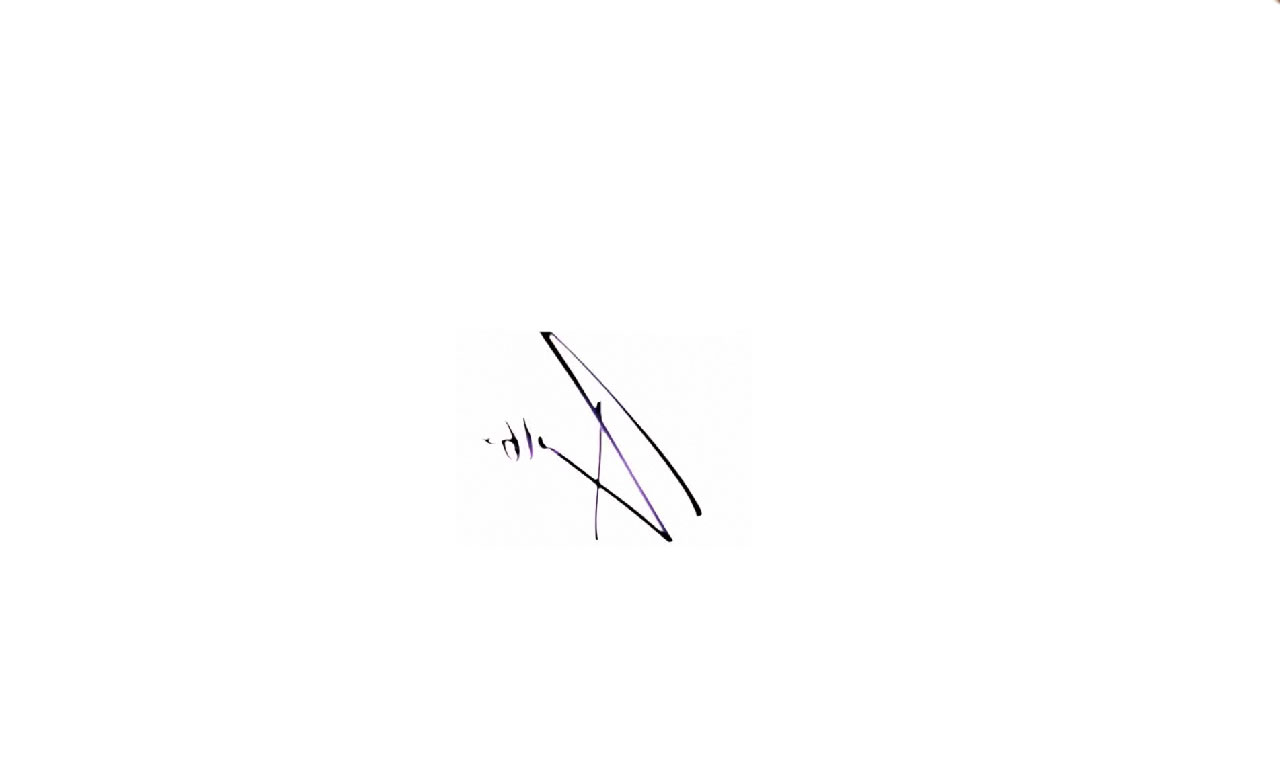The image features a white background with a distinctive scribbled figure positioned in the lower left corner. The scribble is composed of several lines that transition in color from black to purple, changing in both intensity and thickness. It vaguely resembles a complex amalgamation of letters, primarily an 'S' or 'Z' intersecting with a 'P' or 'A'. The structure of these intersecting lines incorporates sharp, angular turns, reminiscent of a broken triangle lacking one side. Adjacent to this intricate shape, there is a vertical line slightly tilted to the left, and further to the left of this line, a dot accompanied by two short vertical stripes. This configuration creates a dynamic visual interplay of lines and shapes against the stark white background.